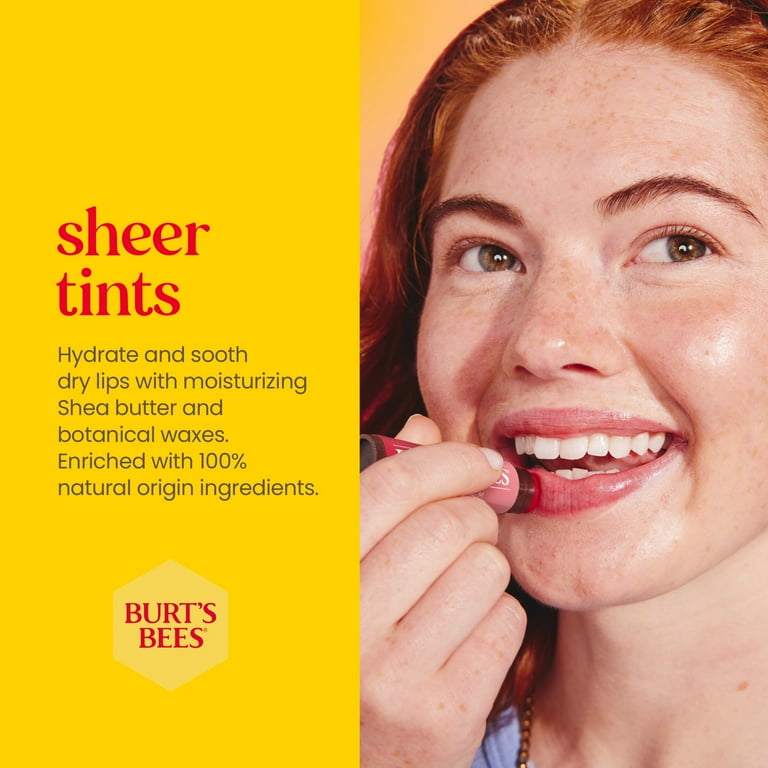This advertisement for Burt's Bees Sheer Tints prominently features a vibrant yellow vertical rectangle on the left side, with attention-grabbing red text at the top announcing "Sheer Tints." Below, in smaller black text, the ad describes the product’s benefits: "Hydrate and soothe dry lips with moisturizing shea butter and botanical waxes, enriched with 100% natural origin ingredients." Further down, a hexagon in a lighter yellow shade contains the brand’s name, "Burt's Bees," in red letters. 

On the right side, a young red-haired woman with hazel eyes and freckles is captured in the act of applying the lip balm to her slightly open, pink-tinted lips, revealing her white teeth in a subtle smile. She holds the product in her right hand, the tube's pink label visible as she gently applies it to her lower lip while glancing to her left. She wears a blue shirt that is barely visible. The ad effectively conveys the promise of hydrated, smooth lips with Burt's Bees Sheer Tints through natural ingredients.